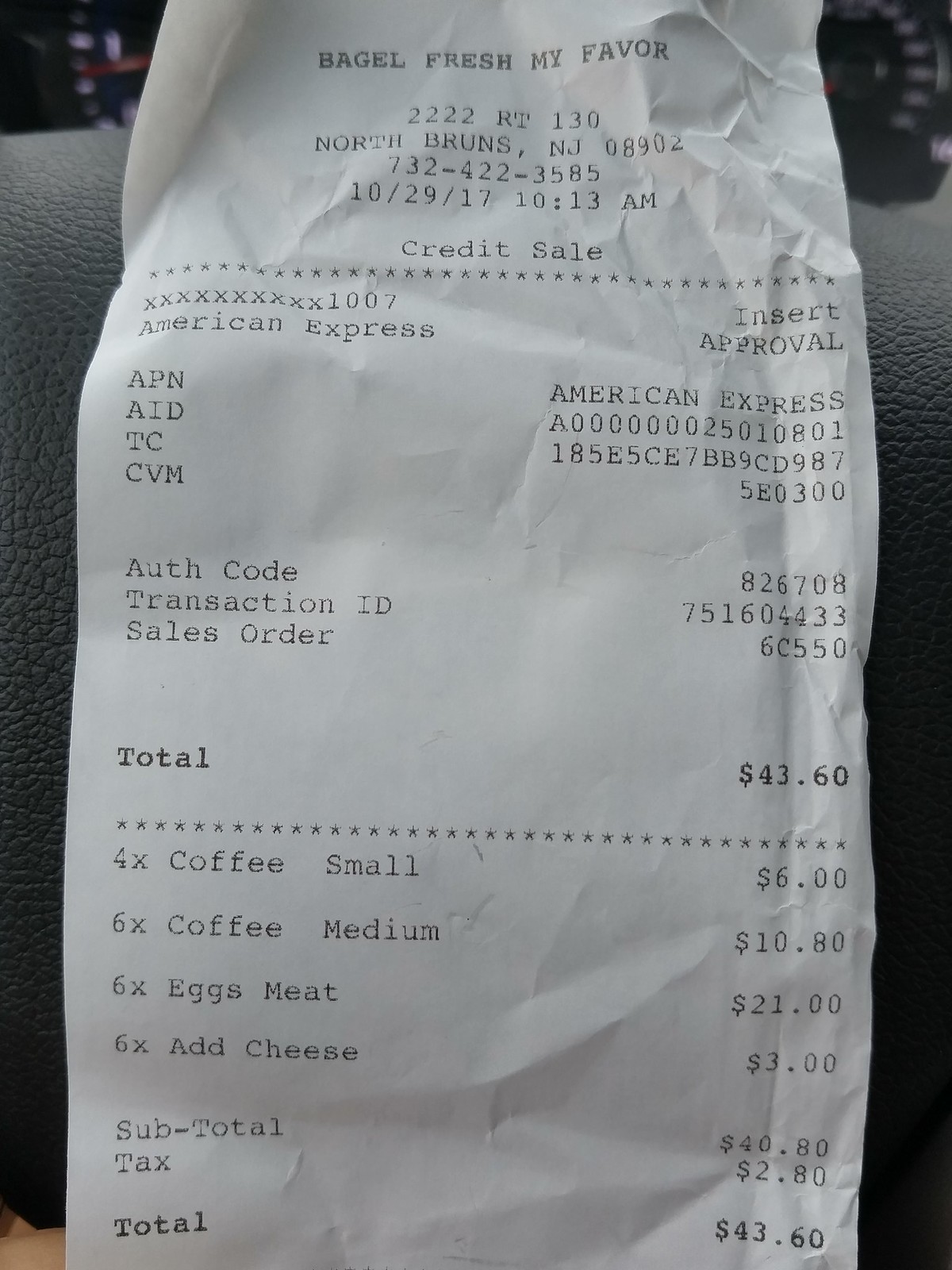Close-up image of a white receipt from a purchase at a coffee shop or bakery called "Bagel Fresh my favor," located in North Brunswick, New Jersey. The transaction took place on October 29, 2017, at 10:13 a.m. The receipt details multiple items including four small coffees, six medium coffees, six eggs, six portions of meat, and six additions of cheese, suggesting the purchase of bagel sandwiches with eggs, meat, and cheese. The total amount spent was $43.60. The image appears to have been taken inside a car, as can be inferred from the blurry, out-of-focus vehicle dashboard and dials visible in the background.